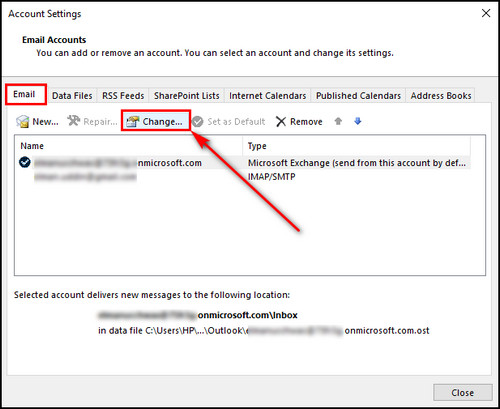The image displays a section of a user interface labeled "Account Settings" in the top-left corner. Below this header, there is a subsection titled "Email Accounts," which offers options to add or remove an email account, or to select an existing account for further configuration. The text and options are presented in black font against a plain white background with subtle gray accents, giving it an unembellished and straightforward look.

Highlighted in red are two key areas: the "Email" text and a "Change" button below it. A red arrow is pointing towards the "Change" button, drawing attention to this option. The image also contains obscured personal information; a name has been blurred out for privacy. The text mentions "Microsoft.com" and "Microsoft Exchange," indicating that these settings are likely managed through Microsoft's email services. Under the "Send from this account by default" instruction, it suggests that selected accounts will deliver new messages to a specified location, though the exact details are partially obscured and difficult to decipher. The interface appears to be part of a corporate or professional email setup, possibly belonging to a Microsoft employee or user.